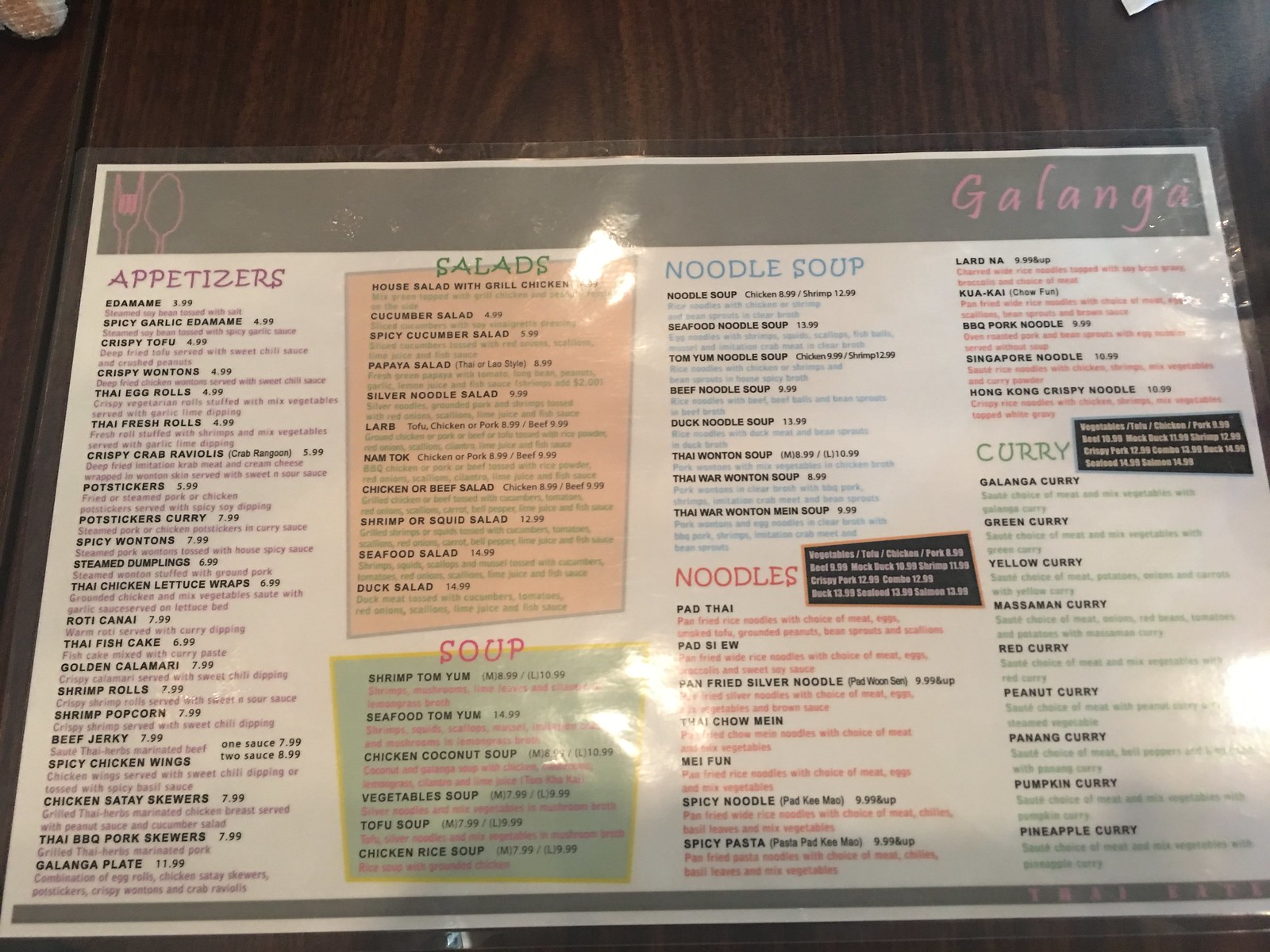This image features a laminated placemat menu placed on a wooden panelled tabletop. At the top of the menu, the restaurant name "Galanga" is displayed in a vibrant pinkish-purple font. Adjacent to the restaurant name is a stylized graphic of a fork making a 'metal horns' gesture, with only the two outer prongs raised and the middle prongs lowered, reminiscent of a rock 'n' roll hand sign. There is also an outline of a spoon complementing the design.

The menu is divided into several sections: Appetizers, Salads, Soup, Noodle Soup, Noodles, and Curry. Each section has a distinct color scheme for easy navigation. The Appetizer section features a purple header with purple descriptions, while the dish names are in black. The Salad section comes with a green header and descriptions, maintaining black font for dish names as well. The Soup section stands out with a green polygon header outlined in yellow, with pink for both its heading and descriptions, and black for dish names. Similarly, the Noodle Soup section uses blue for its header and descriptions, and black for the names. The Noodles section is themed with red headers and descriptions, and black dish names. Lastly, the Curry section mirrors the Salad's color scheme with a green header and descriptions, and black font for the dish names.